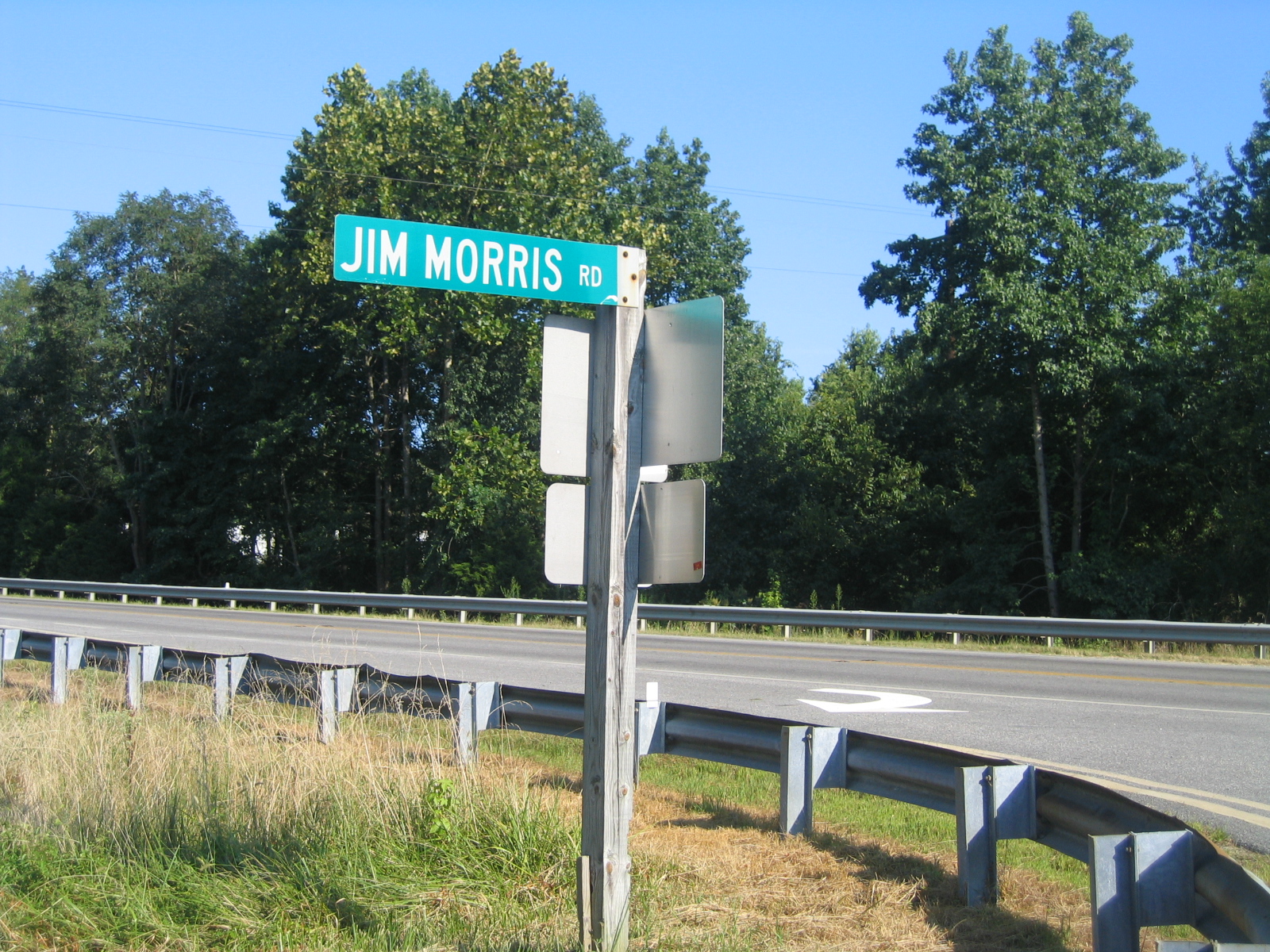A desolate two-lane road cuts through a tranquil landscape in this photo. Prominently positioned in the foreground is a signpost featuring a green street sign with "Jim Morris Road" emblazoned in white letters. Attached to the main signpost are two additional metal signs facing away from the camera, rendering their text unreadable. The lower portion of the image showcases a sandy dirt ground interspersed with sparse patches of weeds, alongside a weathered metal railing that lines the edge of the highway. An arrow sign directs travelers to the right, towards the photo's edge. Beyond the road and railing, a dense cluster of tall green trees sits under a clear blue sky, completing the serene and quiet scene.